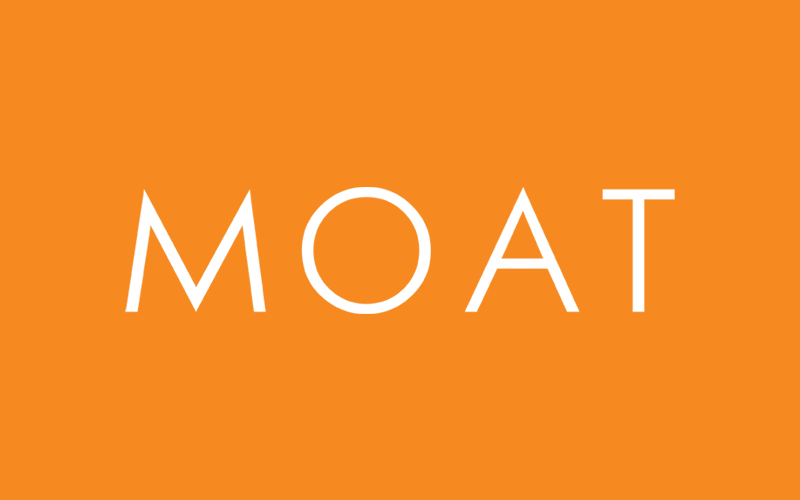The image features a vibrant, pumpkin-like orange background. Dominating the center is the word "MOTE," displayed in large, white capital letters. The font is relatively narrow and takes up about a third of the image's height, with notable spacing between each letter, making the word stand out prominently against the bright backdrop. There are no additional elements or distractions, suggesting that it could be a logo or advertisement for a company, designed to capture attention with its simplicity and bold color contrast.